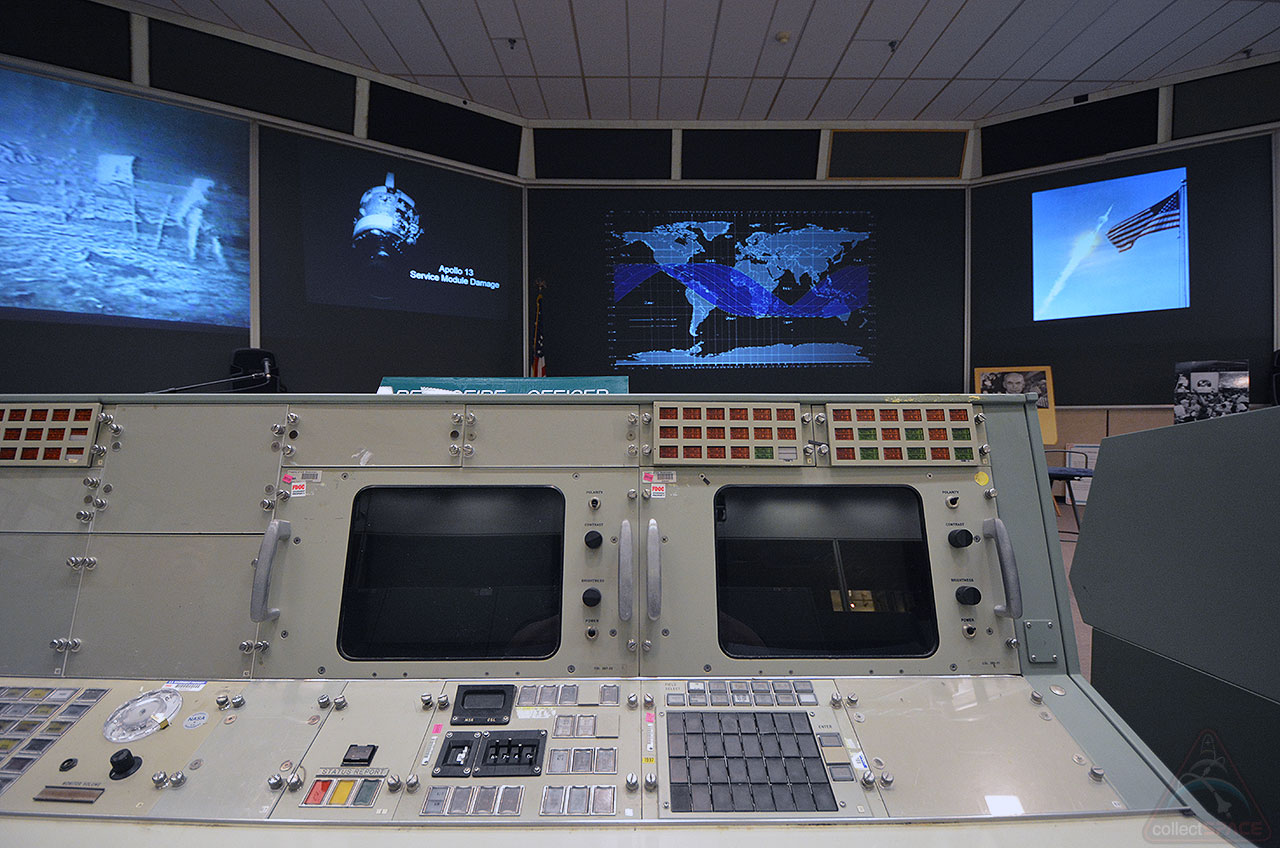The image depicts an intricate setup inside what appears to be a military or space mission control facility, possibly resembling a headquarters or a Pentagon office. At the forefront, there is a control station equipped with two screens and various switches and knobs, currently showing no active displays. Dominating the background are four large screens. One prominently displays a digital map with various coordinates, likely used for strategic operations. Another screen showcases a missile launching adorned with the American flag. A third screen captures an iconic moment of the moon landing, potentially linked to the Apollo missions, and the fourth screen features the trajectory paths of satellites or spaceships orbiting Earth. The overall scene is highly reminiscent of historic mission control rooms from the Apollo era, suggesting a significant link to space missions and operations.